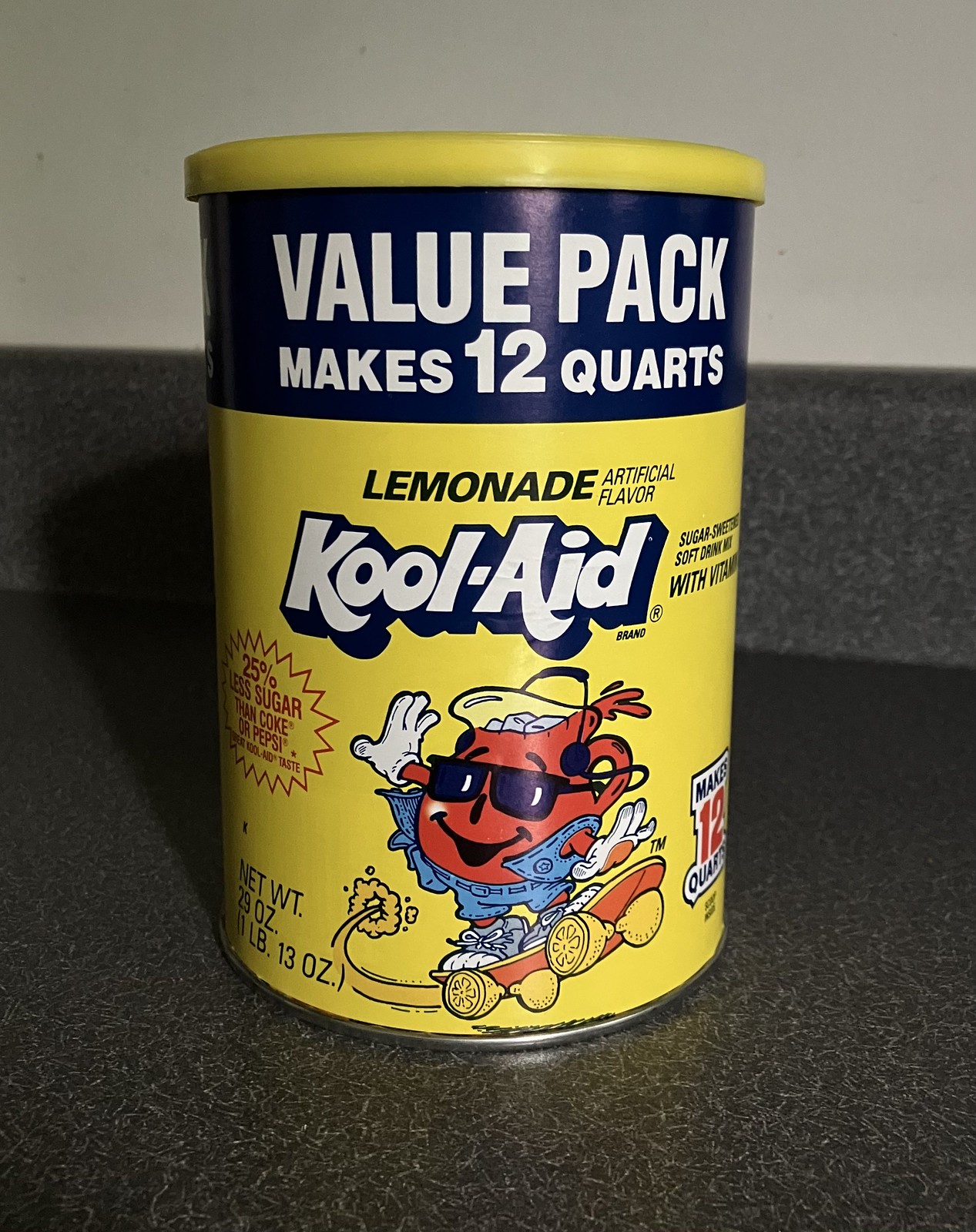This photo depicts a vintage 29-ounce Kool-Aid can, labeled with the lemonade flavor. The can's background is bright yellow, with the word "Kool-Aid" prominently displayed in a white font accentuated by a blue-black shadow. The iconic Kool-Aid Man, a jovial pitcher filled with red Kool-Aid, is featured on the label, riding a skateboard. He sports denim shorts, sneakers, and white gloves, with his arms raised in a triumphant "surfing" pose. Notably, the skateboard's wheels are designed to look like lemons, adding a playful touch. At the top of the can, the label reads "Value Pack."